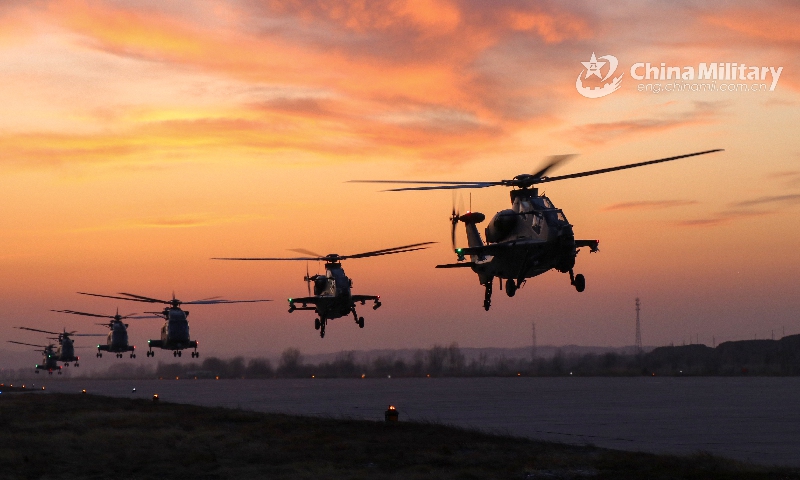In the image, the upper right corner prominently displays the text "China Military." The sky in the background is stunning, painted with a gradient of purple, pink, orange, and gold hues, indicating that it's almost nightfall. A line of six large, dark gray military helicopters dominates the scene, flying across the sky. Below the helicopters, there's a wide strip, flanked by trees on either side and dotted with a couple of light poles and small shining lights in the distance. In the foreground, a few lights dot the landing strip, illuminating the path below. The overall composition portrays a serene yet powerful scene of military air readiness against a beautiful twilight backdrop.